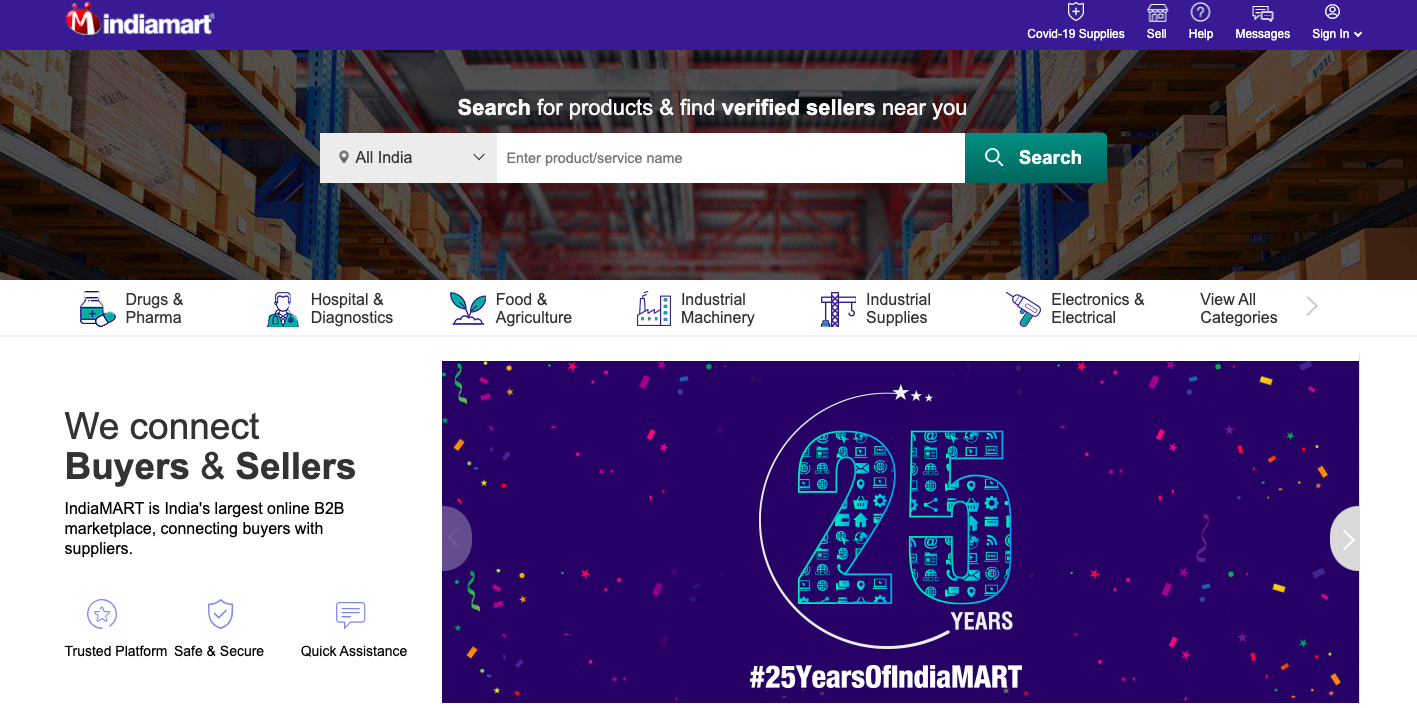In the provided image, there is a screenshot of the India Mart website displayed prominently in the upper left-hand corner. The website's interface shows several navigational buttons in the upper right-hand corner, though they are slightly blurry. The buttons are labeled: COVID-19 Supplies, Sell, Help, Messages, and Sign In.

Below this header, there's a section that invites users to "Search for products and find verified sellers near you." It includes a search bar with the placeholder text, "Enter product/service name." To the left of the search bar, there's a drop-down menu labeled "All India," and to the right of the search bar, a search button is visible.

Subsequently, there's a categorical listing area mentioning various sectors like "Drugs and Pharma," "Hospital and Diagnostics," "Food and Agriculture," "Industrial Machinery," "Industrial Supplies," "Electronics and Electrical," followed by an option to "View All Categories."

Further down, there's a segment promoting the site's services, titled "Reconnect Buyers and Sellers." It states that India Mart is India's largest online B2B marketplace, connecting buyers with suppliers. It highlights features such as "Trusted Platform," "Safe and Secure," and "Quick Assistance."

To the right of this segment, there is an image commemorating "25 years" of India Mart, tagged with "#25YearsOfIndiaMart."